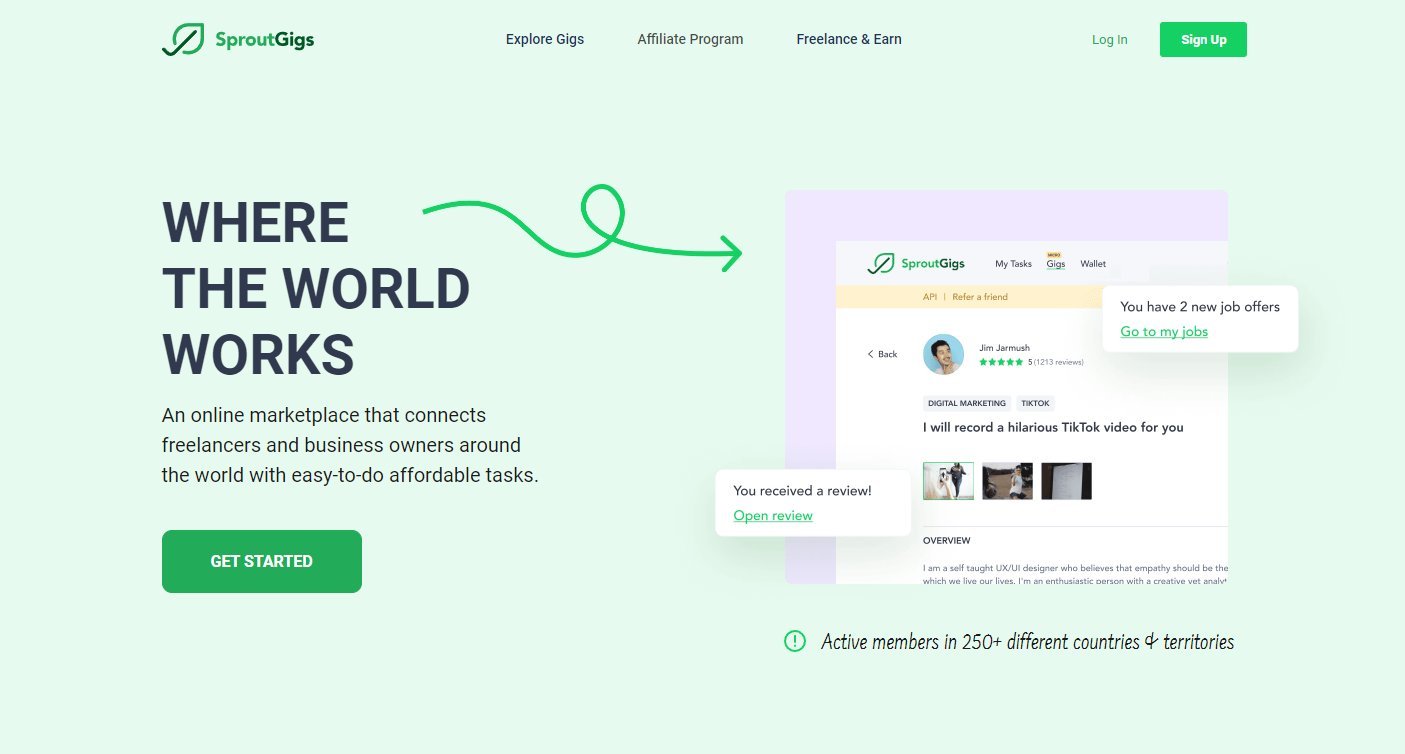**Screenshot of Sprout Gigs Website**

At the top left corner of the screenshot, the text "Sprout Gigs" is prominently displayed. The word "Sprout" is in a lighter green hue, while "Gigs" is in a darker green. Adjacent to this text is a small graphic of a leaf. To the right of this logo, there is a menu in black text featuring options such as "Explore Gigs," "Affiliate Program," and "Freelance and Earn." Further to the right, there are sections for users to either log in or sign up for the service.

Beneath the main navigation bar is a heading that guides users on how to get started with the website. On the left side of this section, a large black font states, "Where the World Works." Below this, in a smaller black font, it explains that this is "An online marketplace that connects freelancers and business owners around the world with easy-to-do affordable tasks."

A prominent green button located below this description reads "Get Started" in white text. A green arrow points from this button to another section of the screenshot, which shows various images of the website in use. These images depict notifications such as "You have two new job offers, go to my jobs," and "You received a review, open review." Additionally, the text highlights that the platform has active members in "250+ different countries and territories."